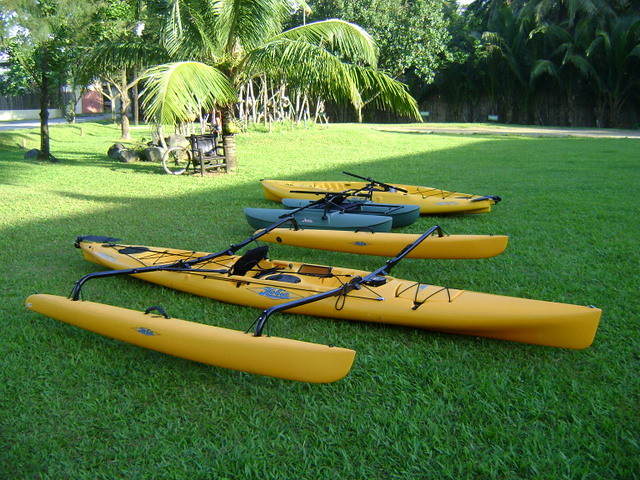This vibrant photograph captures an assortment of kayaks and other paddling crafts meticulously arranged on a lush, green grassy area near a water-based setting adorned with verdant palm trees and tropical plants. Dominating the foreground is a single-person yellow outrigger kayak, distinguishing itself with its stabilizing outriggers and a central seat. Adjacent to this are a sleek, narrow, traditional yellow kayak and a robust, dual-hulled, grayish-blue paddling vessel. The dual-hulled craft, reminiscent of a catamaran with its two pontoon-style hulls, stands out due to its unique design and color contrast. Amidst the grassy expanse, one can glimpse a black chair nestled beneath a palm tree, a nearby bicycle, and an assortment of natural and man-made elements, including a retaining wall, a trailway, and a parking area in the distance. These kayaks, possibly available for rent, enthuse an air of adventure against the scenic backdrop of a tropical paradise.